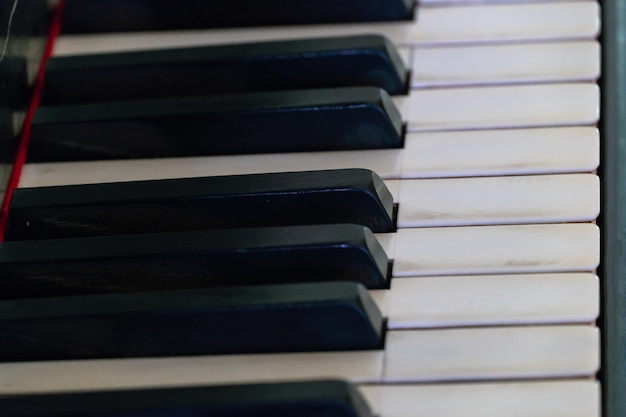The close-up image captures a detailed view of a piano's keys, focusing on nine white and seven black keys. The white keys, which show visible signs of dirt along their edges from frequent use, are positioned toward the right-hand side of the frame. The black keys are seen in groups of twos and threes towards the left-hand side. A thin red line or thread is noticeable running behind the black keys, along with a slightly out-of-focus glimpse of the polished dark brown piano frame. The angle of the shot emphasizes the proximity and arrangement of the keys, highlighting the wear and character of this musical instrument.